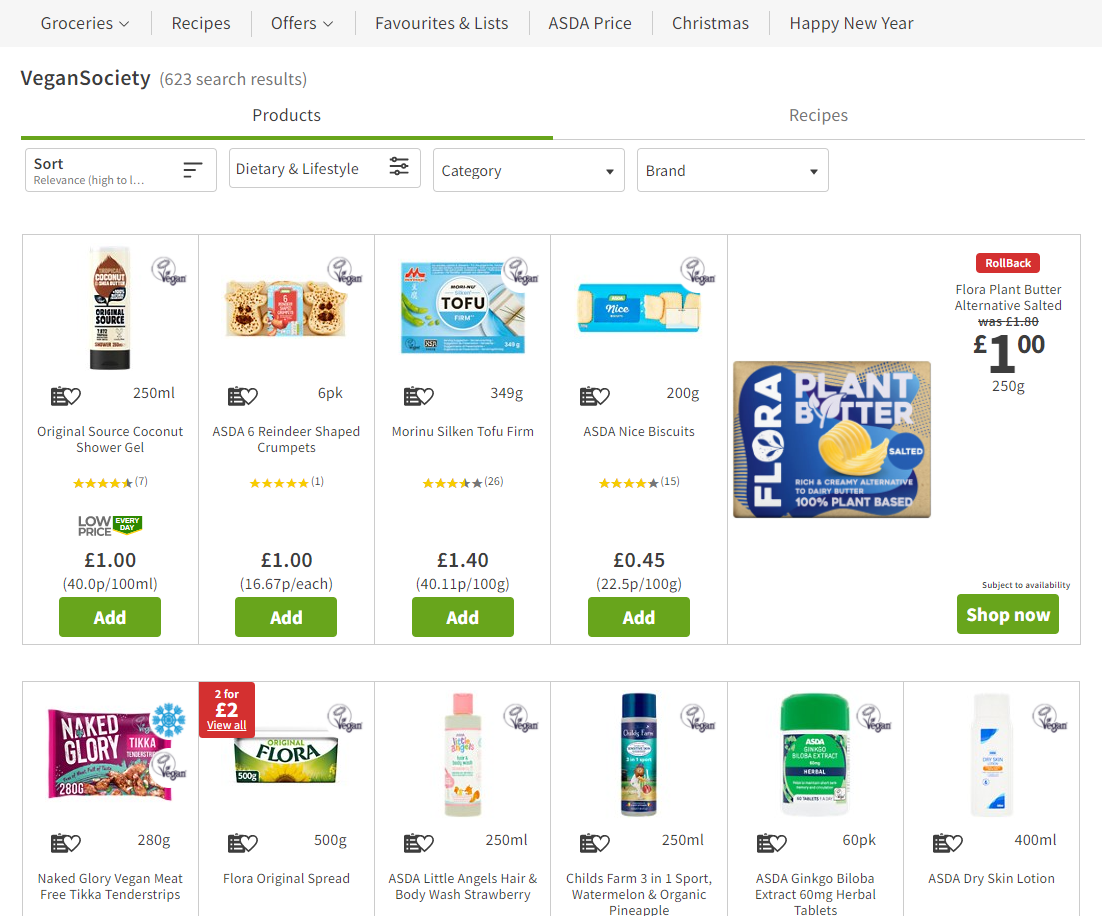### Caption for Grocery Store Web Page Image:

The web page showcases a grocery store with a range of functionalities and products catered to various customer needs. At the top, there is a horizontal navigation bar with tabs labeled: Groceries, Recipes, Offers, Favorites and Lists, ASDA Price, Christmas, and Happy New Year. Below these tabs, the website's name, "Vegan Society," is prominently displayed in dark black ink, followed by a note indicating "623 search results."

Beneath the header, the viewer can toggle between two categories - Products and Recipes. The Products category is currently selected, as denoted by a green line underneath it, while the Recipes category has a thin gray line. Further options for sorting and filtering products by Dietary and Lifestyle preferences, Category, and Brand are available, although it is not immediately clear which, if any, are currently active.

The main section of the page displays four products:
1. **Original Source Coconut Shower Gel (250ml)**: Featured with a product image showing a black base and white bottle. It has an impressive 4.5-star rating based on 7 reviews and is priced at £1 (40.0p/100ml). An option to add the item to the cart is available through a green 'Add' button.
2. **ASDA 6 Reindeer Shaped Crumpets**: Exhibiting a whimsical design with food items creating bear-like faces. This 6-pack has a perfect 5-star rating from 1 review and costs £1, with a unit price of 16.67p each. A green 'Add' button is also present.
3. **Tofu**: Simplified description and price, with an 'Add' button for purchasing.
4. **Biscuits (Cookies)**: Includes a detailed description, price, and consumer reviews, along with an 'Add' button for seamless shopping.

To the right of these products is a larger promotional section featuring **Flora Plant Butter**, accompanied by its image, price, and a prominent 'Shop Now' button.

Below this section, there is a row of six products, each depicted with an image, name, and quantity details:
1. **Naked Glory Vegan Tender Strips**
2. **Flora Original Spread**: A creamy butter-like substance.
3. **Body Wash**
4. **Childs Farm 3 in 1 Support Watermelon and Organic Pineapple Spray**
5. **Abaloba Extract Herbal Tablets**
6. **Skin Lotion**

This detailed layout and product information emphasize a blend of vegan-friendly options and everyday grocery items, making it convenient for customers to browse and shop efficiently.